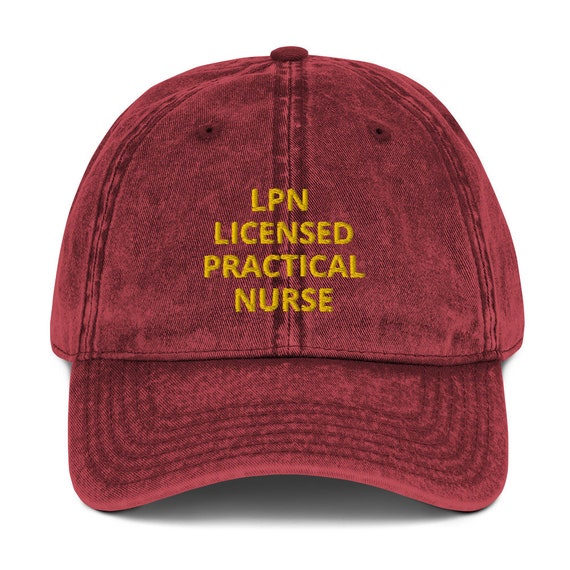This image displays a close-up view of the front side of a baseball cap. The cap, made from a textured fabric, is a deep reddish-brown, often described as burgundy. At the top of the cap is a flat button, and the cap features the typical small air holes and seams that run from the top button down to the sides. The cap lacks internal structure, giving it a more relaxed "dad cap" appearance. Darker, subtly textured lines are present on the bill, signaling careful craftsmanship.

Prominently showcased on the front, the cap has bold, yellow embroidered text arranged in four lines: "LPN," "Licensed," "Practical," and "Nurse," each word aligned directly beneath the previous one. The text is in uppercase letters of consistent size, making the lettering clear and striking against the dark red fabric. The brim of the cap displays curvy stitching lines, adding to the detailed design. Overall, the image captures the intricate details and quality of the baseball cap.